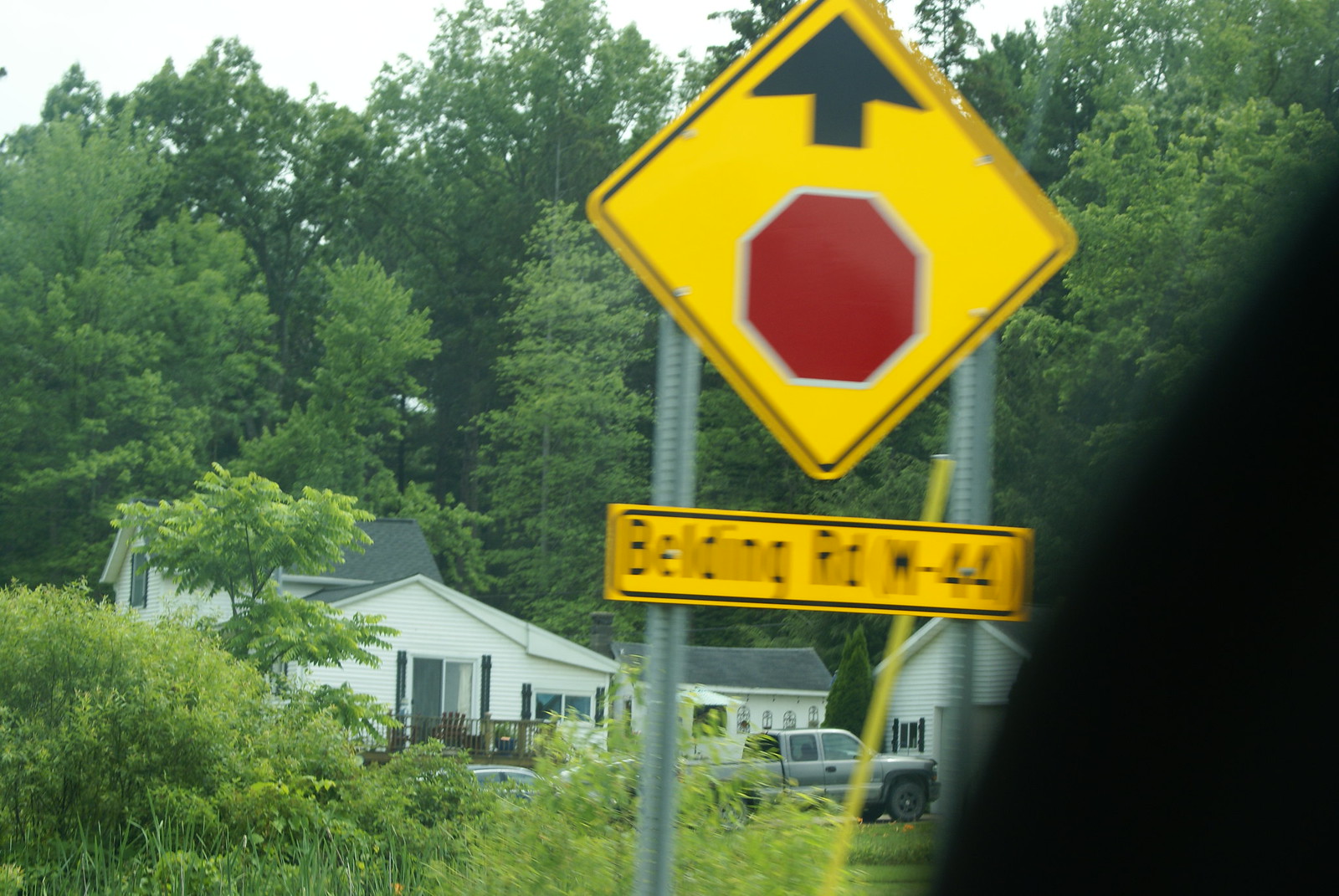In this image of a rural American town, a picturesque forest scene dominates both the background and the foreground with lush green foliage. Nestled amidst the verdant landscape are several quaint houses, adding a touch of humanity to the natural setting. A dark gray truck is prominently visible in the bottom center of the image, parked or perhaps driving along a narrow road that cuts through the greenery. In the forefront, a traffic sign alerts drivers to an upcoming stop sign, with a secondary sign below it indicating "Belding Road, West 44." The sign appears slightly blurry, suggesting the photo was taken from a moving vehicle. Contrasting this, the rest of the image, including the distant houses, trees, and the truck, remains sharp and in focus. In the bottom right corner, a black blotch can be seen, possibly part of the interior of the car from which the photo was taken. The overall scene captures the serene blend of rural life and expansive nature.